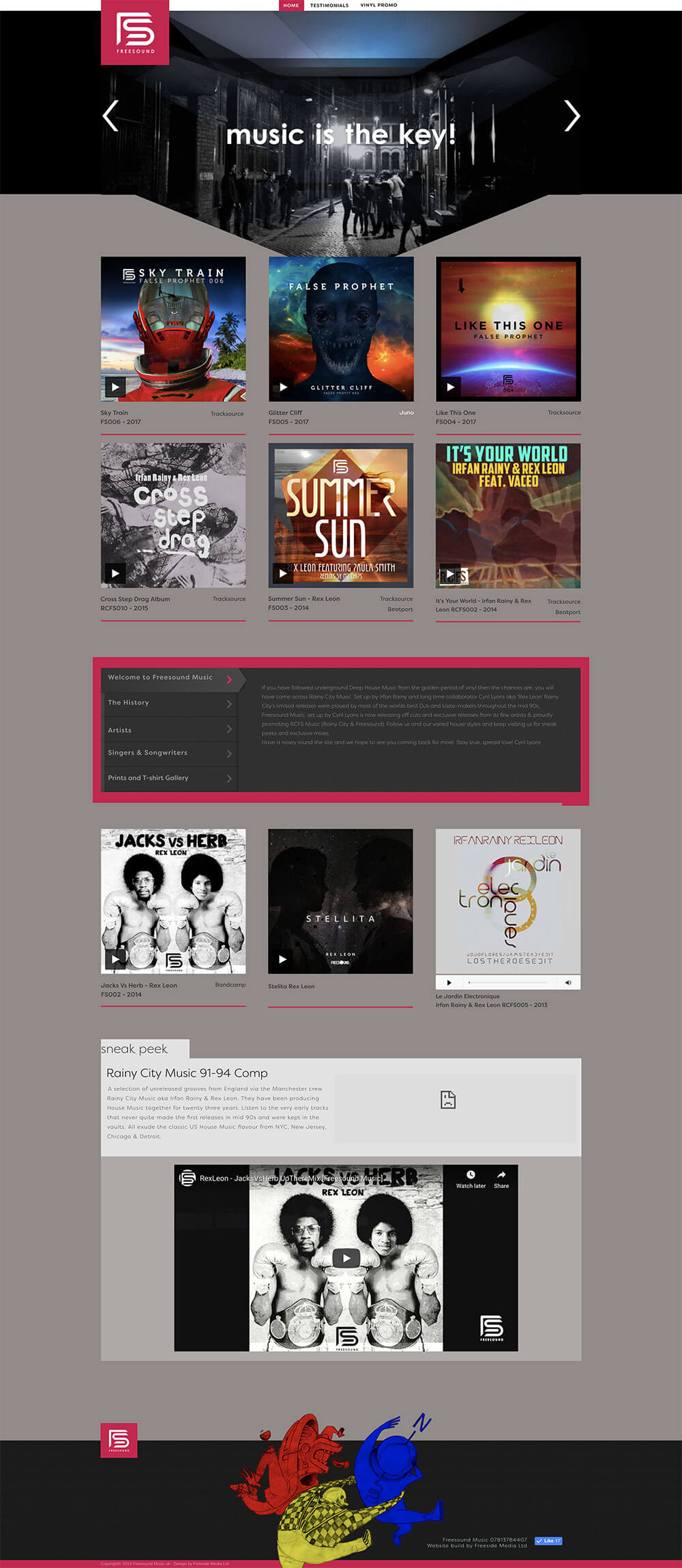In this PlayStation screenshot, the top of the page prominently features the iconic PS icon. The header at the top of the page boldly declares "Music is the Key," set against a backdrop of a black and white photograph depicting several people mingling in the middle.

Beneath the header, the screen showcases six distinct images. The first image includes the text "Something Train" and features a large red structure. The second image carries the theme of "Some Sort of Journey." The third image, though partially illegible, includes a sun. The fourth image is labeled "Cross Step Drag." The fifth image, titled "Summer Sun," displays a pyramid at the top. The final image in this row states "It's Your World."

Below these images, there is a black rectangle framed boldly in red, which contains light gray text that is difficult to decipher. 

Further down, another sequence of three images is displayed. The first of these is a black-and-white photo of two men sporting afros. The middle image is predominantly black with some white lettering, overlaid atop a very blurred white picture. The third image is gray with a stamped "8" imposed on it. 

At the very bottom, there is a repetition of the image featuring the two gentlemen with afros. The footer of the page is black and includes an icon representing dancing people, highlighted in red, blue, and yellow.